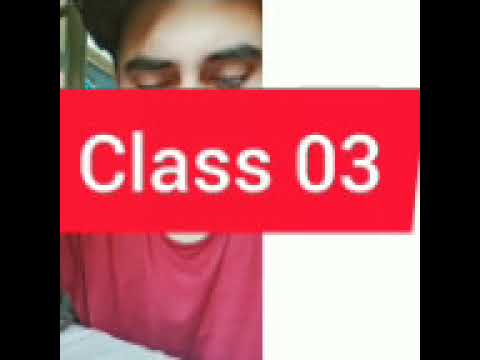The image features a vibrant red horizontal banner stretching across the center, inscribed with "Class 03" in white letters. The "C" is capitalized, while the other letters are lowercase. Behind the banner on the left side is a close-up of a young man's face, visible from his eyebrows upward. His eyes appear closed, suggesting he might be blinking or looking down. His face is partially shadowed on the upper left side, contrasting with the brightness on the rest of his forehead. He has dark brown eyebrows and eyelashes, with dark hair peeking out from the upper left corner. Below the banner, his maroon shirt is visible, along with a sliver of skin beneath his neck, resting above a white surface in front of him. The image is flanked by black vertical bars on both the left and right sides, taking up about 10% of the image width each, with the right 40% dominated by a white vertical section.